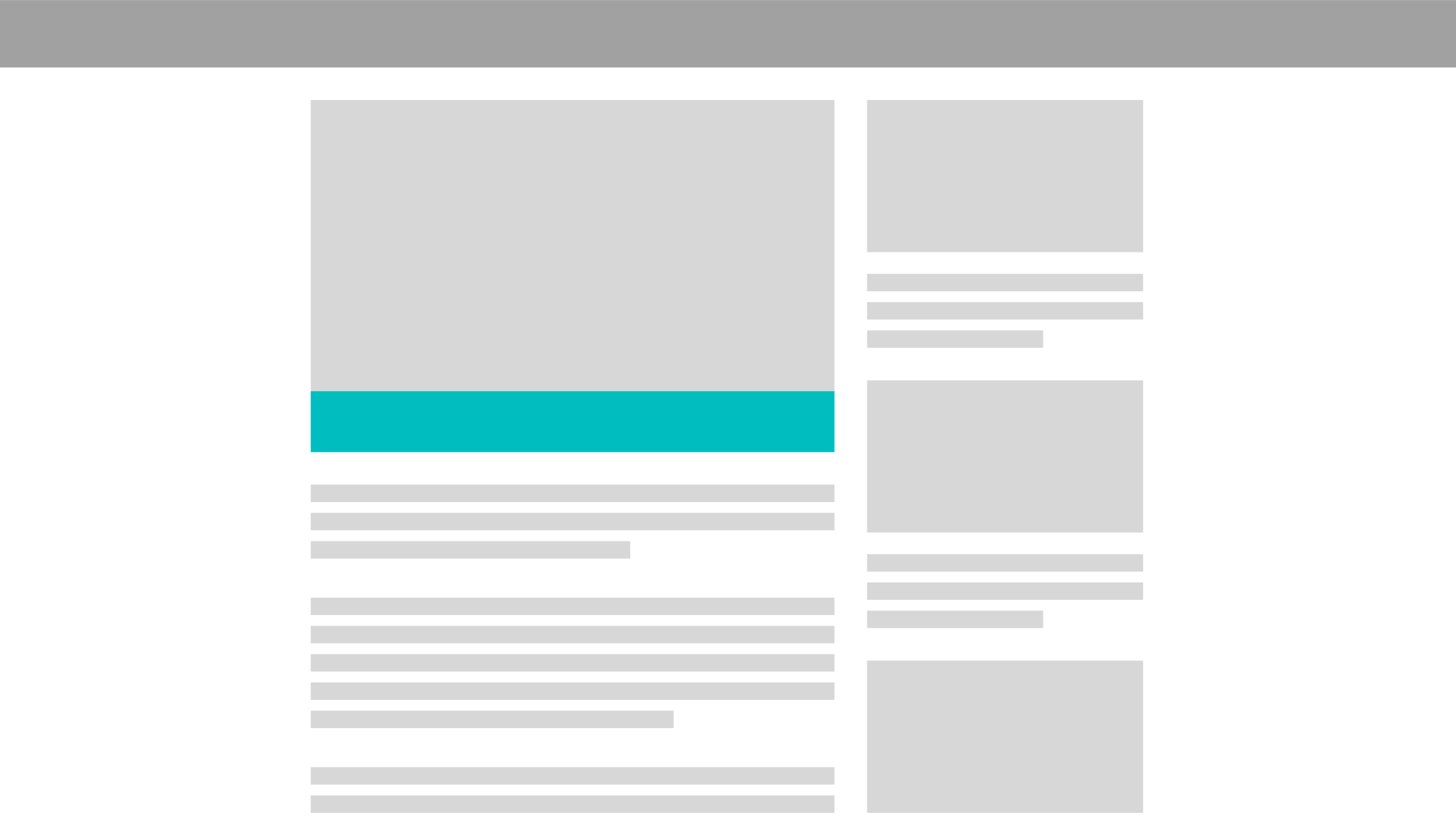This screenshot depicts an empty website template with a white background. At the top of the image, there is a wide gray horizontal rectangle that likely serves as the banner area for navigation links. Beneath this, on the left side, there is a larger gray rectangle which appears to be a placeholder for a photo. Attached directly below this image placeholder is a smaller blue rectangle, likely intended as a label or caption for the photo.

Further down the layout, there are ten thin gray rectangles placed in a vertical sequence, which seem to represent consecutive lines of text perhaps for a description or article following the image.

To the right of this arrangement, at the top of the section, there is another standalone gray rectangle that might function as another image or heading. Below this, there are three thin rectangles stacked vertically, also likely representing lines of text. This pattern repeats with another larger gray rectangle, then three more thin text lines, followed by one more larger gray rectangle at the bottom. This visually structured placeholder template seems poised for further content integration, providing an orderly space for images and text placement on a website.